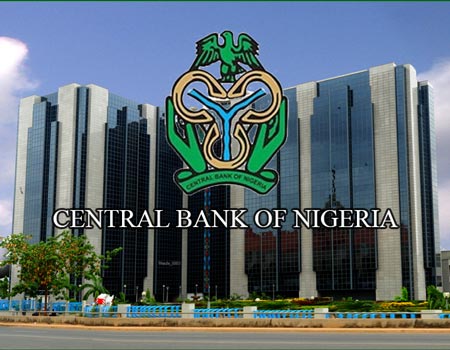This photograph captures a towering, approximately 20-story multi-story office building identified as the Central Bank of Nigeria. Dominating the center of the image, the building features large glass windows segmented by tan or off-white stripes. The base of the image hints at a highway or road, with some greenery including trees and bushes visible in the foreground. The blue sky and clouds form a serene backdrop. Overlaid on the photograph is the Central Bank of Nigeria's emblem and name; the name is written in capital letters with a thin, blocky white font. The logo, positioned above the text, is intricate, featuring three gold or yellow horseshoes aligned to create a blue "Y" in the center. This configuration is cradled by two green hands, topped by a green eagle with wings outstretched, symbolizing protection and authority. The image appears to have been taken during the daytime from a street-level perspective, capturing both the grand architecture of the building and the clear, bright sky above.